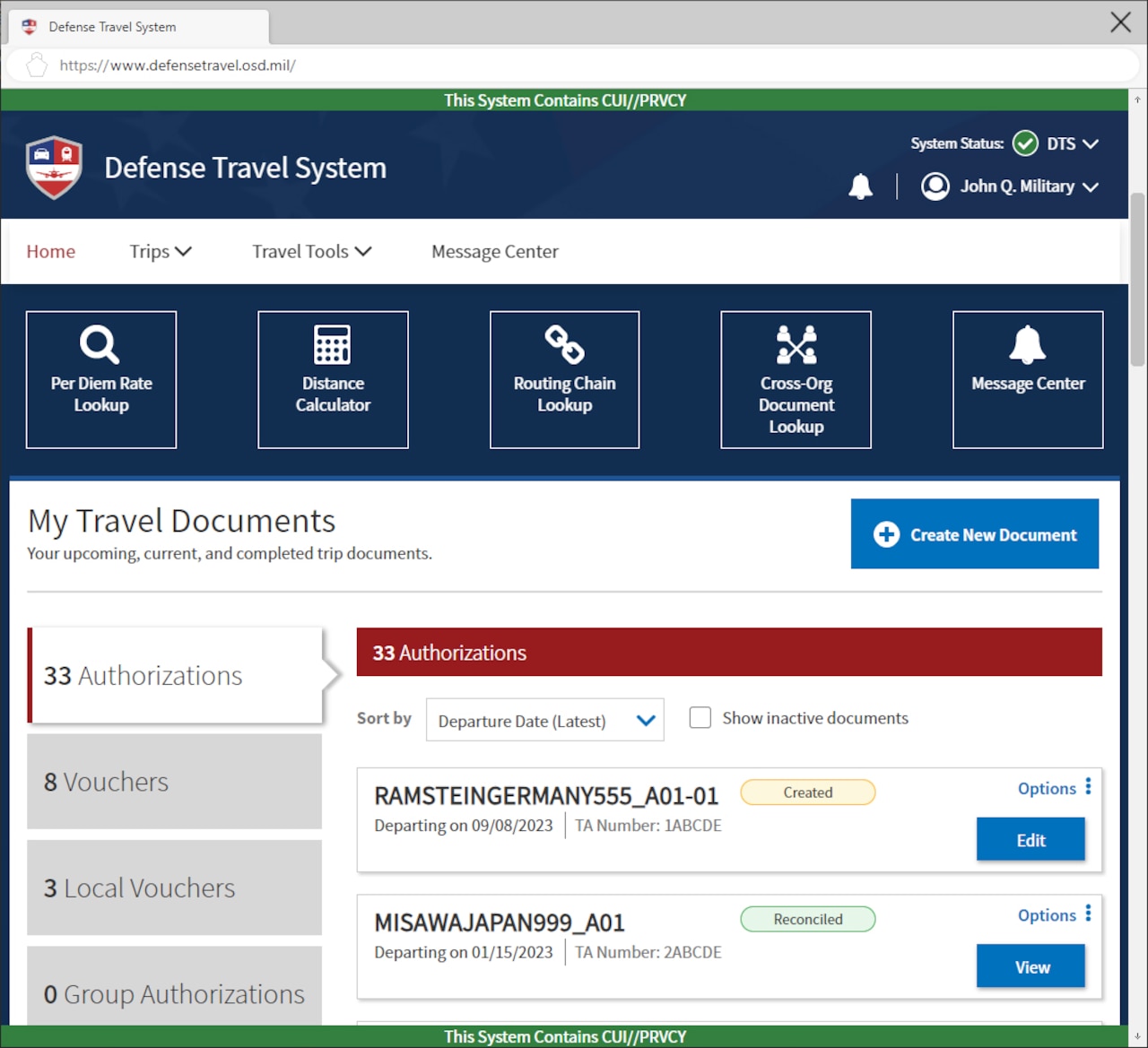A detailed screenshot of the Defense Travel System's (DTS) dashboard interface is presented, specifically showing the Foreign National Travel (FON) system found at the URL www.defensetravel.osd.mil. The system contains Controlled Unclassified Information (CUI), indicated by the acronym "PRVCY," symbolizing privacy. The system status is denoted by a white checkmark inside a green circle.

The main navigation bar includes several tabs: "Home," highlighted in red, and "Trips," "Travel Tools," and "Message Center," all in black. Key tools listed under "Travel Tools" include PRDOM Rate Lookup, Distance Calculator, Routing Chain Lookup, Cross Org Document Lookup, and Message Center.

On the right side of the interface, there is a section titled "My Travel Documents" that categorizes documents into upcoming, current, and completed trips. On the left panel, detailed statistics are provided: 33 authorizations, 8 vouchers, 3 local vouchers, and 0 group authorizations.

At the top of the dashboard, a blue rectangle prominently features a button labeled "+ Create New Document." Additionally, a notification symbol appears next to the user name "John Q. Military," highlighting alerts within the Defense Travel System.